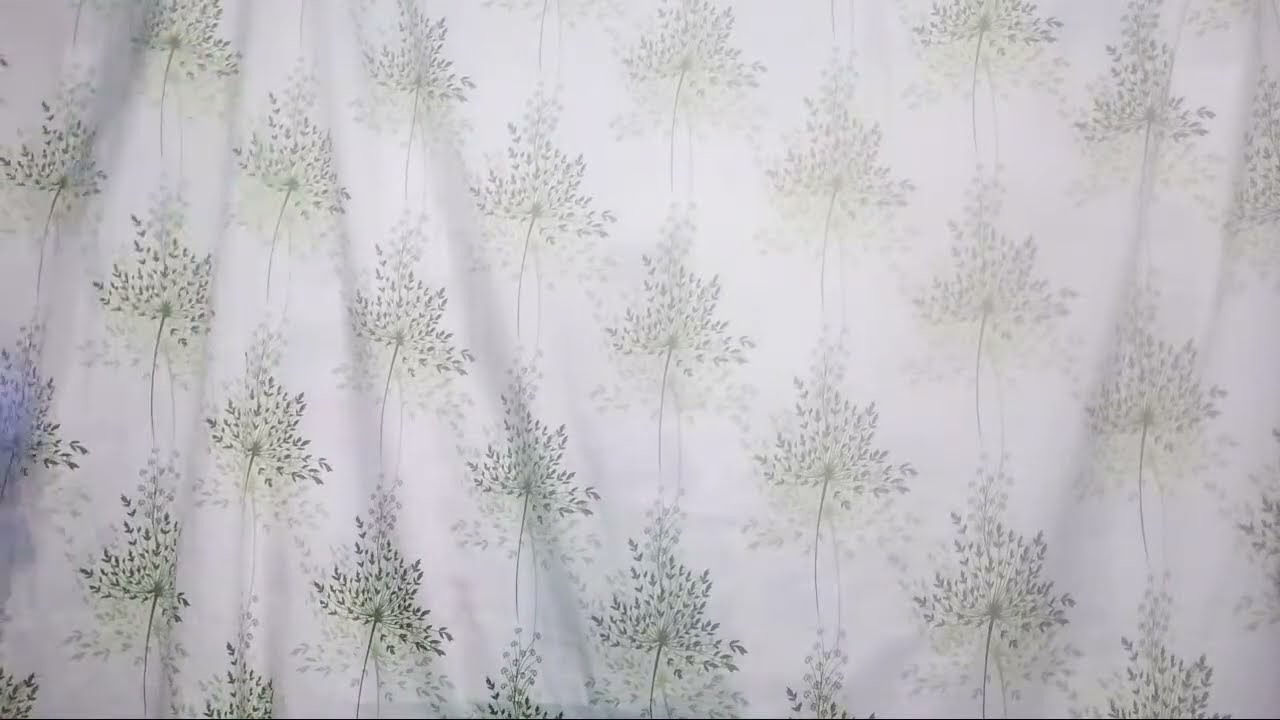The image captures a flat surface, possibly a piece of fabric like a shower curtain or bed sheet, positioned directly in front of the camera at a distance of 4 to 5 feet. The background is a light gray to white color, featuring a repetitive print design that includes diagonally aligned rows of stylized trees or tree-like flowers. Each small tree consists of a thin vertical stem with clusters of gray foliage sprouting from the top. The rows are arranged so that each upper row is interposed in the gaps of the row below it, creating a harmonious and symmetrical pattern. There are also thin, spindly shadows overlaying the surface, reminiscent of tree branches. Additionally, the surface shows subtle wrinkles or ruffles, confirming the material could be fabric.